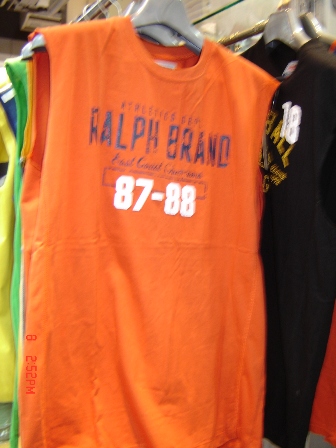The image depicts a vibrant orange tank top, prominently displayed on a clothing rack. The sleeveless shirt features the brand name "Ralph Brand" emblazoned in bold blue lettering across the front. Directly beneath the brand name, the numbers "87-88" are written in clean white text. Surrounding the main garment, similar clothing items are partly visible; immediately behind the orange tank top is a sleeveless green shirt of a similar style. To the right of the main focus, a black T-shirt is positioned, facing towards the left side of the image, adding depth to the scene. The array of apparel hints at a diverse and organized display, emphasizing the orange tank top as the centerpiece.